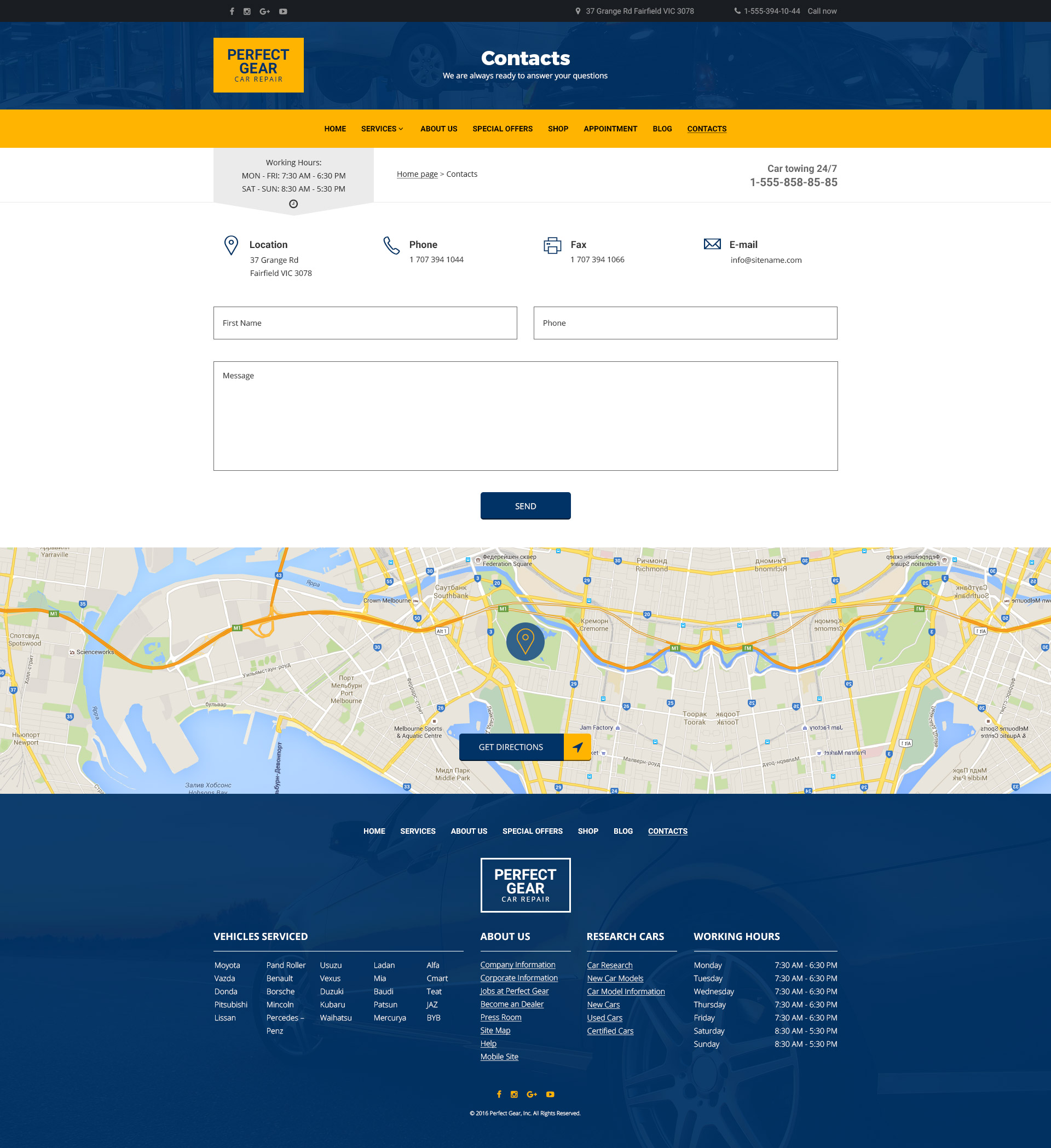A screenshot of a contact form is displayed at the top of the image, featuring fields labeled for first and last names (although the text is too small to be read clearly). Below the fields, there is a light blue 'Send' button. Taking up most of the midsection, there is an embedded Google Map displaying various geographical elements: blue rivers, tan-colored dirt patches, and a complex network of orange lines denoting roads in multiple directions. Towards the bottom, text entries indicate different sections or links for user navigation, including "Perfect Gear," "Vehicle Serviced," "About Us," "Research Cars," and "Working Hours."